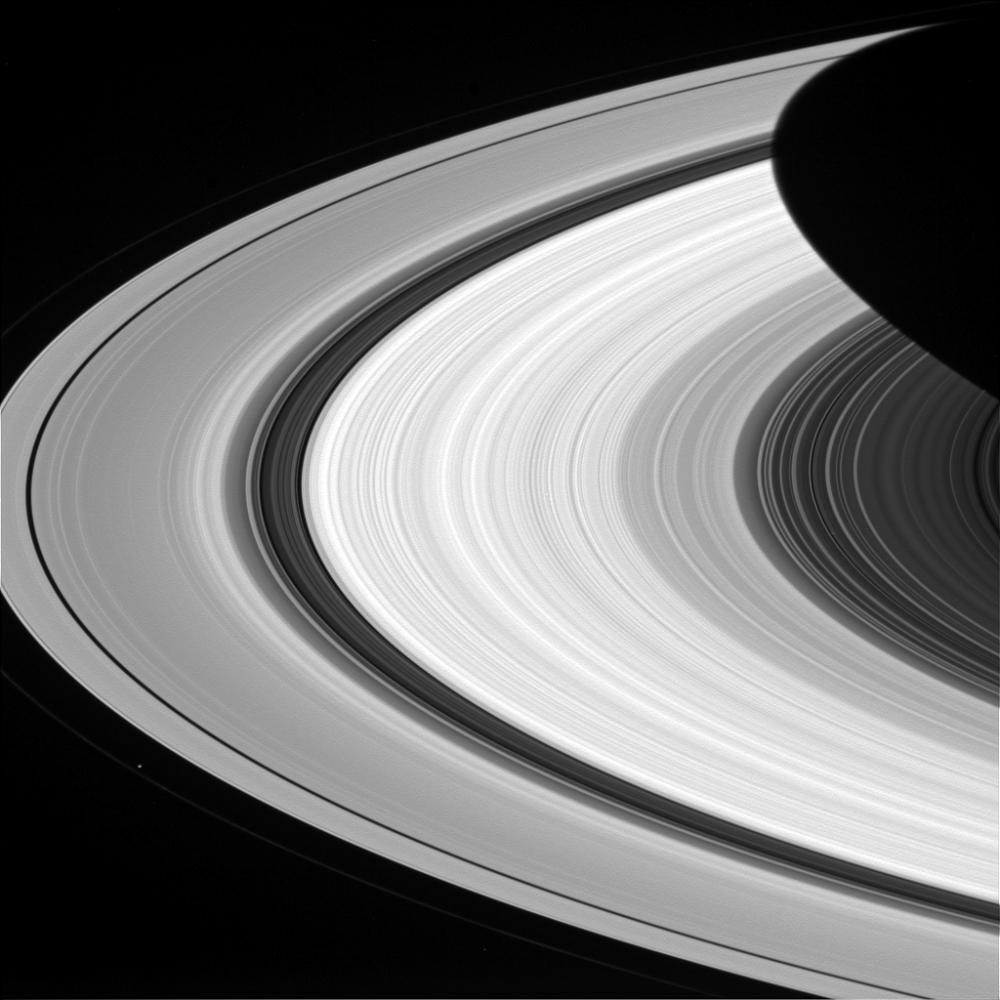This detailed black-and-white image is enigmatic and open to various interpretations. Set against a completely black background, it prominently features a series of concentric rings that evoke the look of planetary rings, such as those of Saturn, or the grooves of a vinyl record. The rings emanate from the left side of the image, leading towards the center, which is partially obscured in the top right by a shadow or darkened blob.

The rings exhibit a gradient of shades, starting from an outermost thin gray ring, followed by a narrow black ring. The gradient continues with bands transitioning from gray to white, back to a darker gray, then to lighter gray again, eventually leading to darker shades of gray and black. These bands vary in width, with some narrow and others wider, creating a dynamic visual texture.

Towards the center, the rings get narrower and darker, contrasting sharply with the lighter colors towards the outer bands. Despite the lack of color, the intricate gradation from black to gray to white adds depth and complexity to the image. The exact nature of the image remains ambiguous, leaving viewers to wonder whether it is a photograph, a close-up of a tangible object, or an abstract illustration.